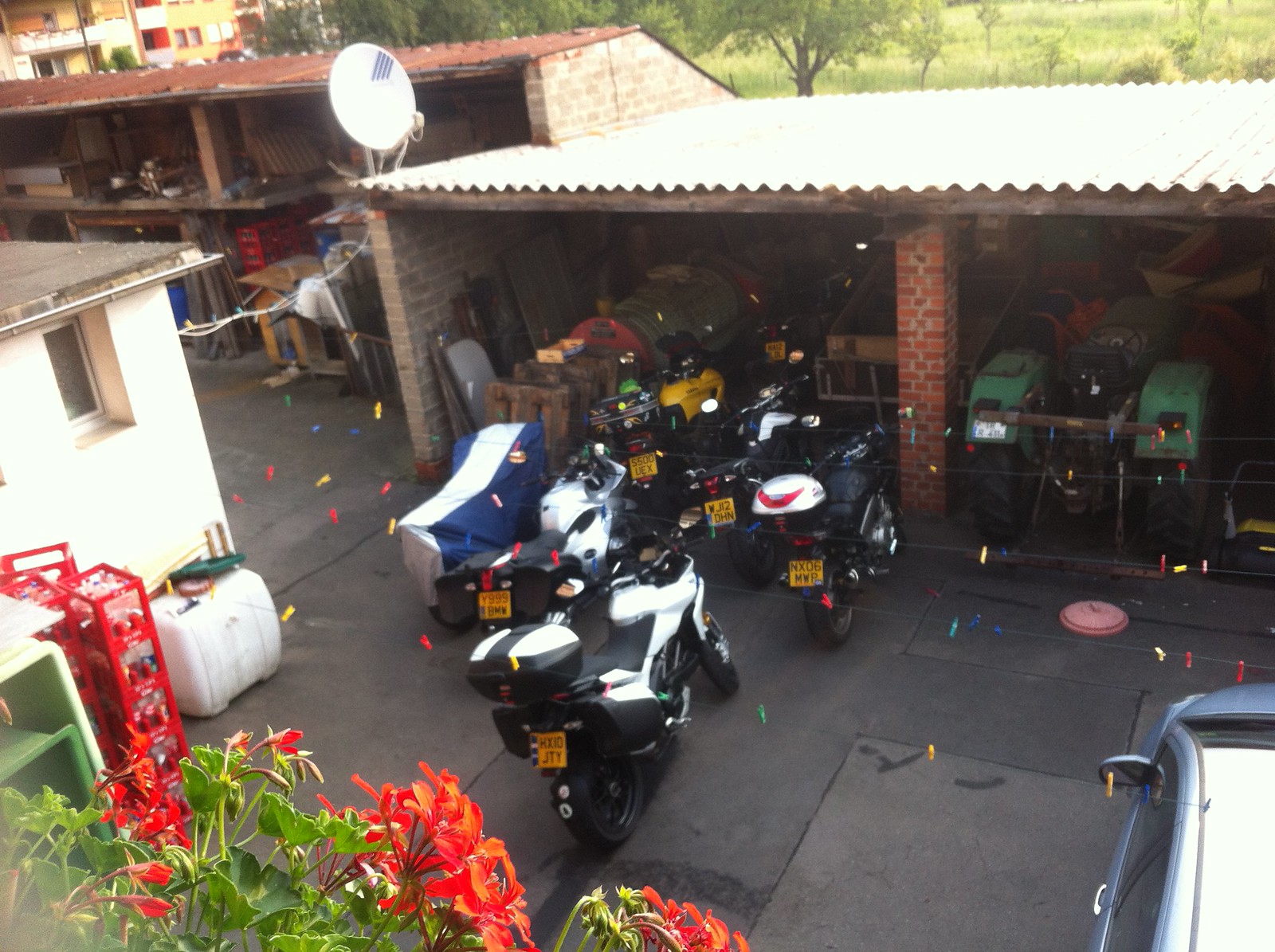In this high-angle photograph taken from a rooftop, the main focus is an open garage made of simple brick walls and a tin metal roof. Inside the garage, seven motorcycles are neatly lined up, three of which spill out onto the dark gray, tiled or tarred surface in front. The motorcycles display a variety of colors including black, gray, silver, black and white, and blue and white—all with yellow license plates. The garage appears to adjoin another brick and metal roof storage building. Adjacent to the motorcycles, there is a very old green tractor within another section of the garage. 

To the left of the garage stands a squat house with deep inset windows and white walls. The foreground of the image showcases vibrant red flowers with green leaves. In the bottom left corner, there are crates of drinks, a white container, and a green and white shelf. Meanwhile, on the bottom right, the edge of a light blue car is visible. Additionally, a yellow flat object can be seen towards the top left, and trees with grass create a natural backdrop to the scene. A satellite dish is placed atop one of the buildings further adding to the setting.